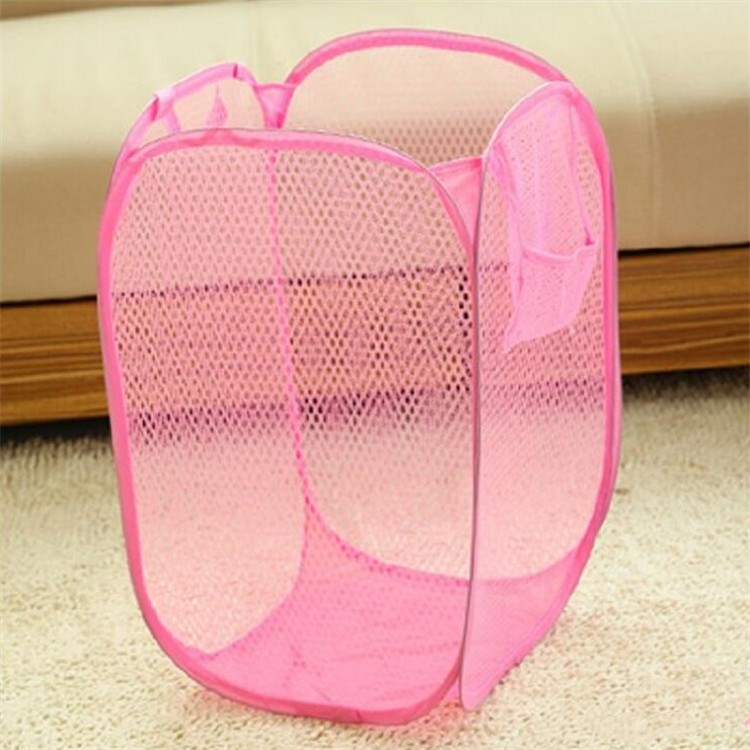The photograph showcases a hot pink collapsible laundry hamper. Made from thin mesh and wire, this rectangular-shaped hamper features rounded edges and is designed to fold in half by pushing one side inward. The mesh body includes a small net pocket on the right side for accessories, and it has two hot pink handles for easy carrying. The hamper is set on a beige or tan carpeted floor, and a wooden running board is visible behind it. In the background, there's a piece of furniture with a wooden frame, likely a sofa, with beige-colored cushions that more or less match the carpet. The scene is evenly lit, indicative of indoor lighting from above, and the photograph itself is square in dimensions.